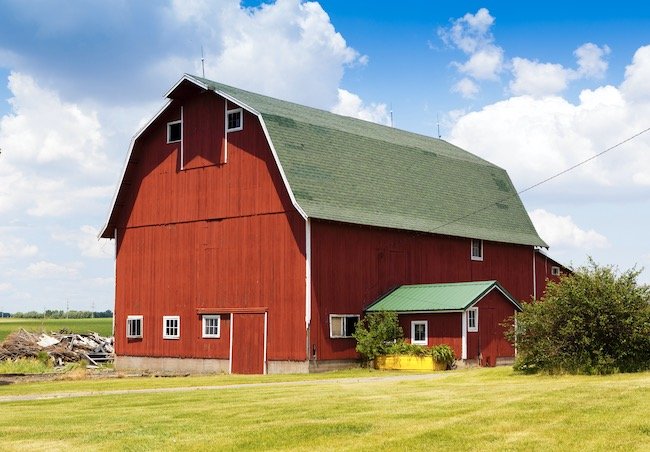This daytime photo captures a striking red barn situated on an expansive, flat grassy landscape. The barn features a freshly painted red wooden exterior with a subtly contrasting gray roof. Prominently visible are three white-framed windows at the bottom, and an additional two windows positioned near the top. The barn also boasts a red door and an awning over the front entrance. 

Attached to the main structure, there is a smaller add-on building with a green roof and several windows, extending slightly to the side and back, creating an interesting architectural profile. Surrounding the barn, the ground is covered in a mix of freshly mowed but slightly yellowing grass. 

To the left of the barn, there is a noticeable pile of old wood and assorted junk, contributing to the rural ambiance. A road or pathway leads up to the barn, hinting at regular use of the structure. On the far right, a sizable green shrub is present alongside a green planter filled with various plants, adding a touch of vibrant greenery to the scene. Above, white and gray clouds drift across an expansive blue sky, completing this picturesque farmhouse setting.